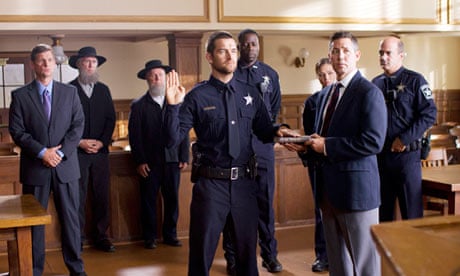In this detailed color photograph, a solemn courtroom scene unfolds as a law enforcement officer, likely in his forties, takes an oath. Standing at the front of the courtroom, the officer dons a navy blue uniform adorned with a star badge on his chest. His short-cropped hair and raised right hand highlight the seriousness of the moment, while his left hand rests on a Bible held by a gentleman in a navy blue suit. The man in the suit looks forward, possibly towards a judge whose position is indicated by the corner of a brown desk visible in the upper right of the image.

Behind the central figures, a diverse group of individuals adds depth and context to the scene. To the right, standing slightly behind the officer, are two more law enforcement officials. One is a tall Black gentleman, and beside him is a shorter female officer, both observing the proceedings with focused attention. Further back, a bald-headed middle-aged man stands next to them. On the left side of the courtroom, another man in a suit appears attentive, marking the area where the defense and prosecution tables are visible.

At the back of the courtroom, near the spectator's gallery, two men dressed in distinctive dark suits and wide-brimmed black hats, resembling Amish attire, stand out with their large beards and solemn expressions. Another man in a colored suit positions himself in front of them, adding to the tableau of this meticulously captured moment of judicial and communal significance. The room itself, with its wooden seating and white walls, wraps the scene in a traditional courtroom ambiance.